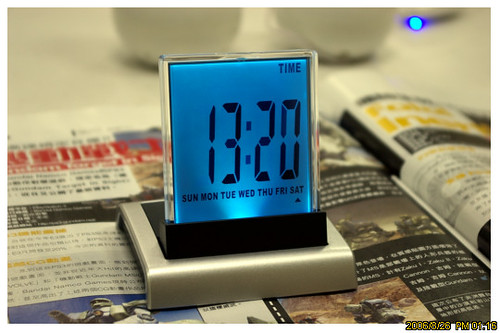A sleek, modern clock takes center stage in this image, perched atop a magazine with Asian characters on its cover, which is laid on a table. The clock itself is encased in a clear, square-like structure made of plastic or glass, and is mounted in a holder that blends a striking contrast of black and silver. The background features a metallic, luminous blue, adding an ambient glow to the scene. The digital display of the clock reads "13:20," indicating the time is 1:20 PM. Below the time, the days of the week are listed in an abbreviated format: SUN, MON, TUE, WED, THU, FRI, SAT. A small, blue triangle underlines "SAT," signifying that it is Saturday. This sophisticated timepiece seamlessly combines functionality with modern design.